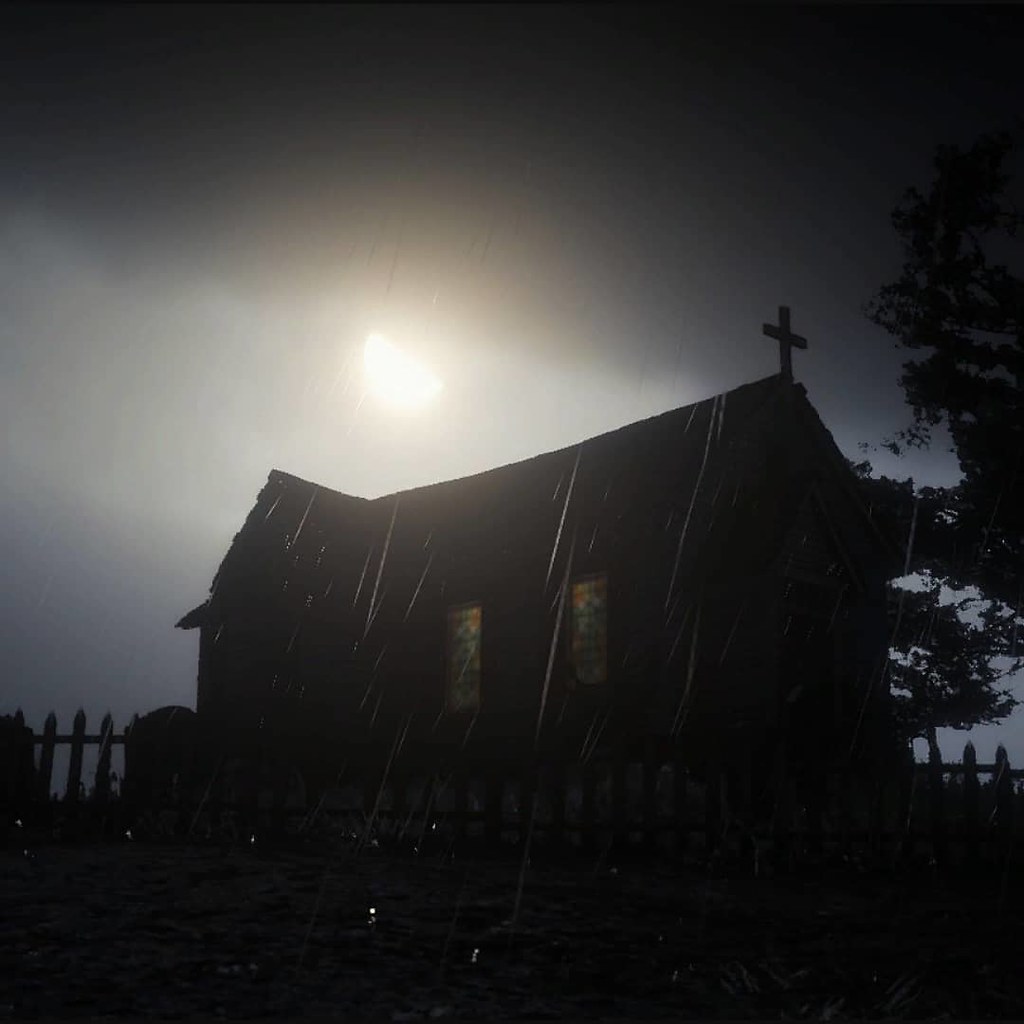In this dark, silhouetted image, a church stands prominently as the central subject, identifiable by the large cross crowning its rooftop and its distinctive stained glass windows, though the colors are subdued due to the low light. Surrounding the church is a picket fence, mostly visible on the sides. The scene appears to be set during a rainy night, with streaks of rain illuminated by the moonlight that filters through dark clouds, creating a backlit effect. To the right of the church, one or possibly two trees are silhouetted against the night sky, adding to the overall spooky and somber ambiance of the image. The moonlight enhances the eerie atmosphere, casting an otherworldly glow over the entire scene.